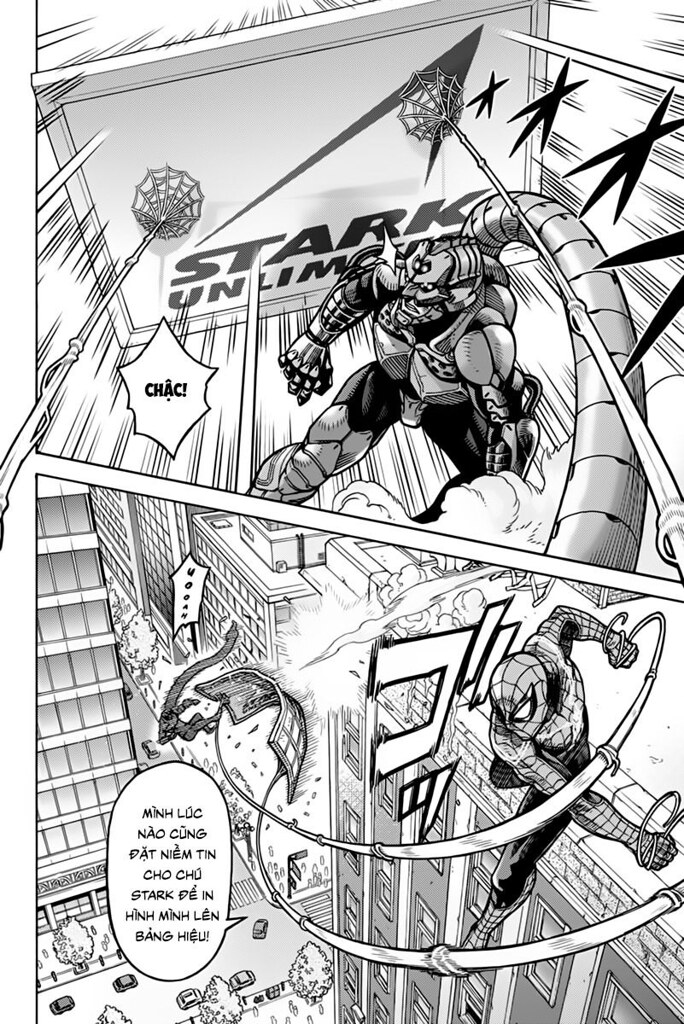This vertical rectangular image in black and white captures two dynamic cartoon scenes separated by a diagonal line. At the top, above a cityscape that appears to be downtown Manhattan, the phrase "Stark Unlimited" is prominently displayed, indicating a connection to Tony Stark. Spider-Man's webs can be seen, suggesting his residence at a high vantage point. Meanwhile, another character, possibly a villain like Green Goblin, is present. The bottom image showcases Spider-Man mid-action, seemingly throwing an adversary off a building. Both scenes are set against the backdrop of tall buildings with windows and a brick apartment structure, emphasizing a bustling city environment. The entire piece is filled with intense action and excitement, and the dialogue bubbles are written in Vietnamese, indicating the comic's multilingual accessibility.